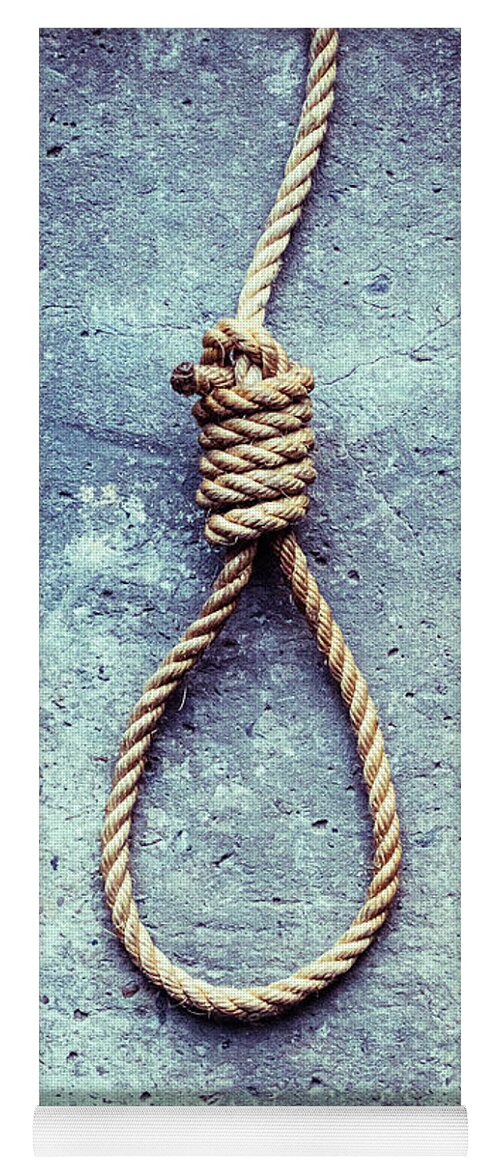The image depicts a vertically oriented noose made of a thick, helically wrapped rope. The noose lies on a concrete surface with a distinctive bluish tint, illuminated by a light source above. The structure of the noose shows five coils, and the rope extends upward, suggesting it is secured at the top. The bottom part of the image includes a holder, most likely plastic, which helps position the photo on a white surface with a white background.